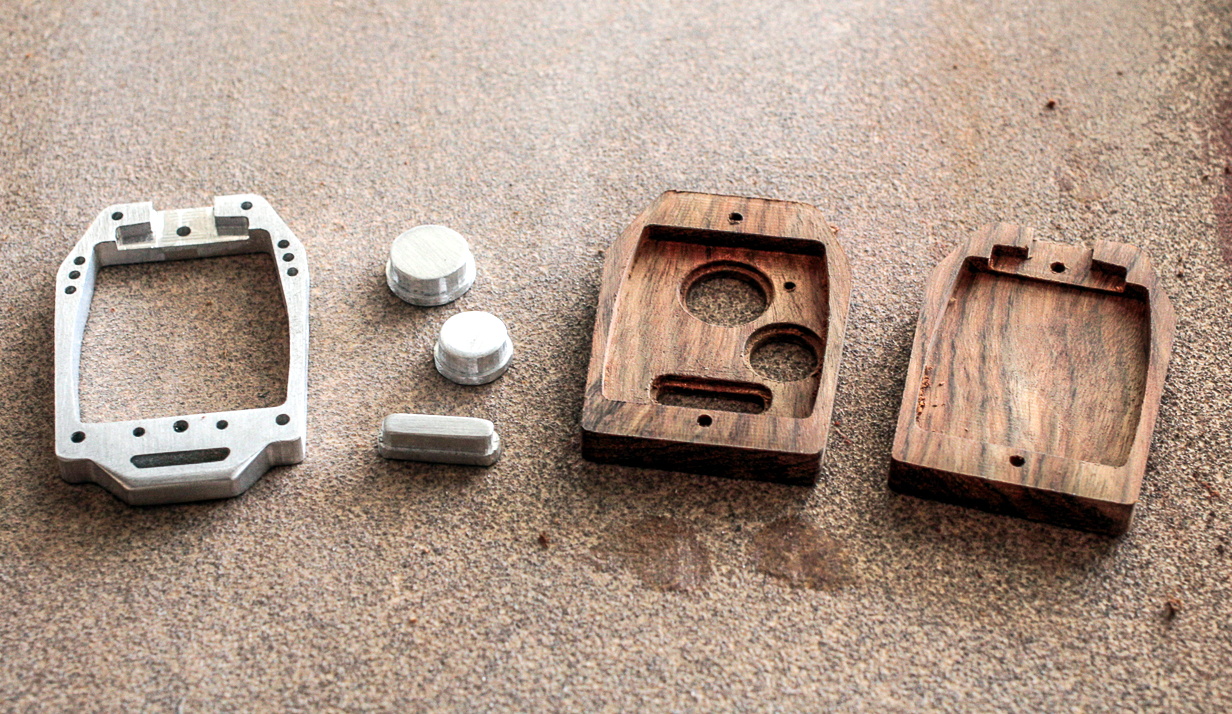The image features dismantled parts of a mechanical device laid out on a textured, grainy metal surface sprinkled with bits of dirt. Central to the scene are two large wooden panels, one of which is square with multiple drilled holes and indentations, suggestive of puzzle pieces fitting into a larger construct. The second wooden panel, located to the left of the first, has one prominent large hole, two smaller ones, and an oblong cutout. Accompanying these wooden pieces are three metal knobs—two round and one oblong—positioned between a large, singular metal piece and the wooden panels. The large metal piece seems to complement the other components with its purpose likely involving those knobs, aiding in the assembly of the device. The overall placement and design of the parts imply they are machined to interlock, contributing to an intricate mechanical system once assembled.